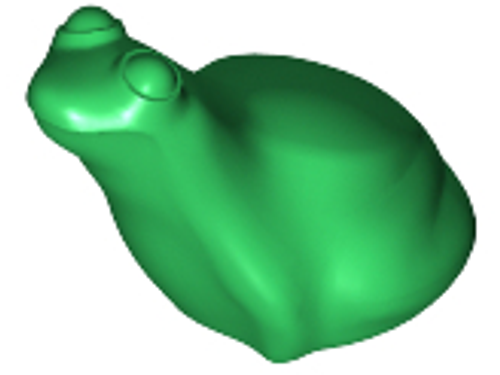The image is of a green, frog-shaped figurine that appears to be made out of plastic and possibly digitally altered or 3D printed. The frog has a rounded, legless body with a noticeable back hump and is positioned facing the left. Its eyes are bulbous and located on the top of its head, with no pupils or intricate detailing. The frog's mouth is a faintly curved indent, giving minimal facial detail. The green color of the figurine is shiny and varies in shade, with a darker green on the top due to shadowing and a lighter green on the front. The background is plain white, adding to the slightly pixelated and blurry appearance that resembles a CAD drawing or a simple children's toy depiction.